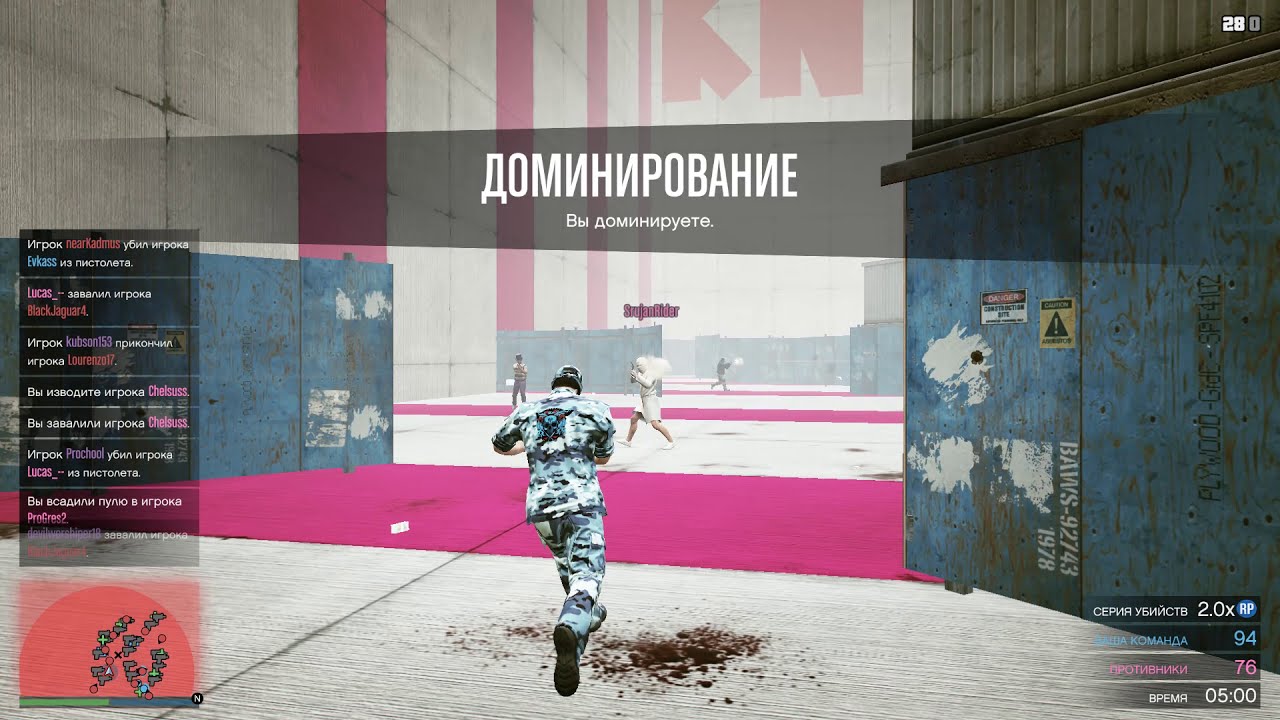The screenshot depicts a third-person shooter video game featuring a player character clad in camouflage clothing, running forward through a massive industrial building with his back turned to the camera. The concrete floor beneath his feet has vibrant pink stripes across a gray base and noticeable blood splatters, suggesting recent combat. Overhead, there is text in Russian set within a gray rectangle near the top edge of the image. To the left, you can see a menu panel with different options and at the bottom, a small map indicating the player's position in the game. Various other characters are visible in the background, engaged in different actions. The walls, made of weathered plywood and metal, enclose the scene, while the flooring transitions into areas with the pink hue. The image also includes a UI element displaying numbers "2.0X" and "94, 76," adding to the game's interface.